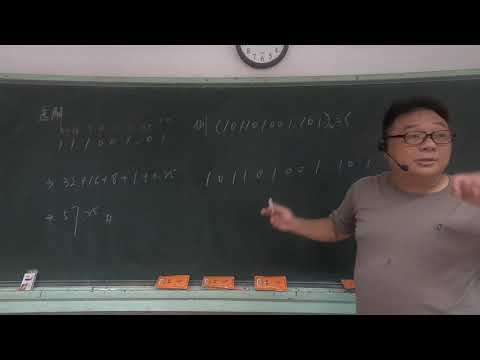A middle-aged Asian man with short black hair and dark-framed glasses is standing in front of a green chalkboard, captured mid-speech. He wears a tan t-shirt and a headset with a microphone positioned over his right ear. His right hand holds a piece of chalk, which he is using to gesture toward the chalkboard filled with mathematical formulas and equations. His left hand is raised, further emphasizing his explanation. The chalkboard also features three visible orange-backing erasers at the bottom and a partially visible clock above it. The man appears to have an inquisitive expression as he looks toward his audience. This scene is framed by a black banner on the top and bottom, suggesting the image might be displayed on a computer screen.